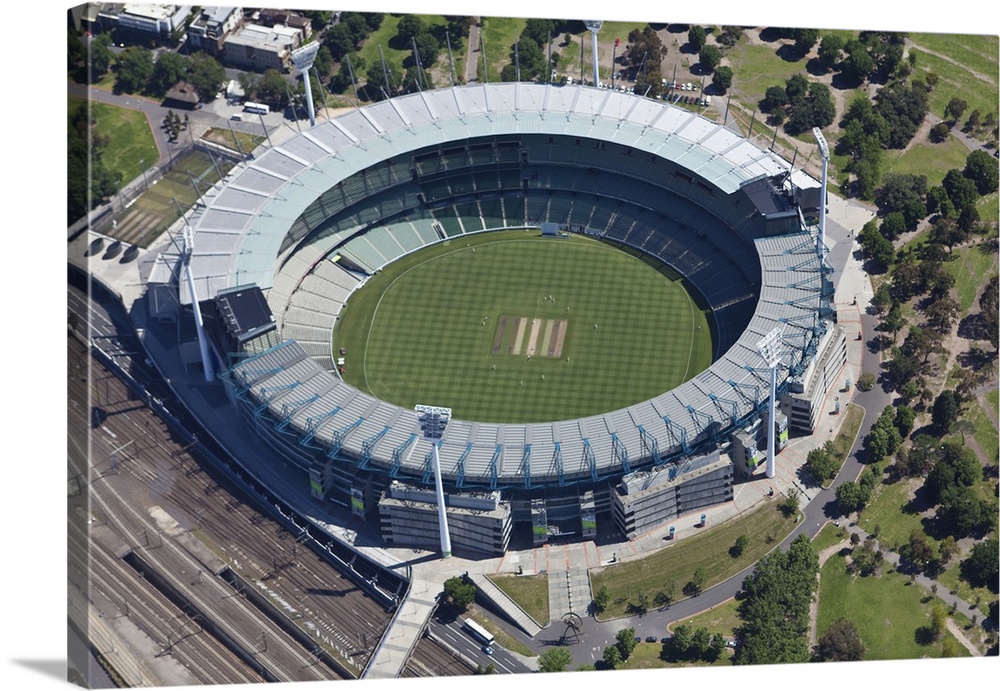This detailed aerial image captures a circular blue stadium surrounded by vibrant green grass at its center. Encircling the stadium, varied green trees of different sizes create a diverse and lush landscape. Bushes are situated closer to the street, highlighting the dense greenery. A well-maintained, silver-gray road cuts diagonally across the bottom left-hand corner of the image. The scene is brightly lit by daylight, underscoring the outdoor setting. The image also features stadium lights and additional grassy fields and trees around the stadium, with a highway visible nearby.